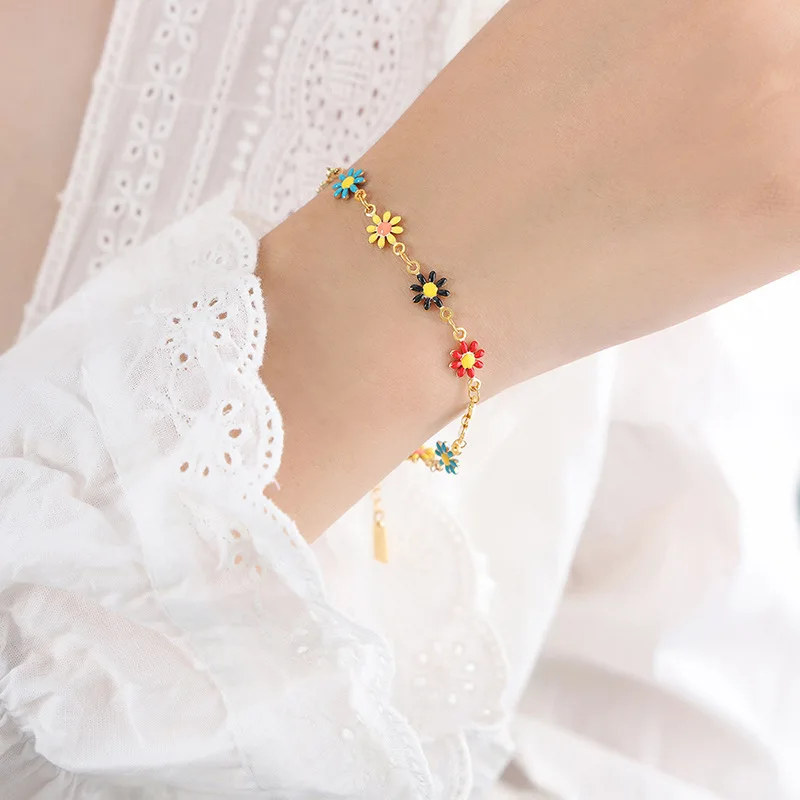This color photograph, in a portrait orientation, captures a detailed and vibrant image of a woman modeling an exquisite bracelet. The woman, with her porcelain white, youthful skin, is adorned in a flowing white dress with an embroidered scalloped edge and a flared ruffle design at the cuff. The dress, consistent in its delicate white embroidery, extends to a partially visible shoulder and a hint of her chest.

The focus of the photograph is a fine gold chain bracelet draped elegantly on her wrist, which enters the image diagonally from the bottom left corner to the top right. The bracelet features five identically shaped enamel daisies, each in a different color, meticulously detailed from top to bottom: an aqua daisy with a yellow center, a yellow daisy with a pink center, a black daisy with a yellow center, a red daisy with a yellow center, and a blue daisy with a yellow center. The vibrant colors of the bracelet's flowers are accentuated by the white backdrop, making them pop vividly and drawing significant attention to the jewelry. This photograph exemplifies realistic product photography, with a strong emphasis on the bracelet's intricate design and the elegance of its presentation.